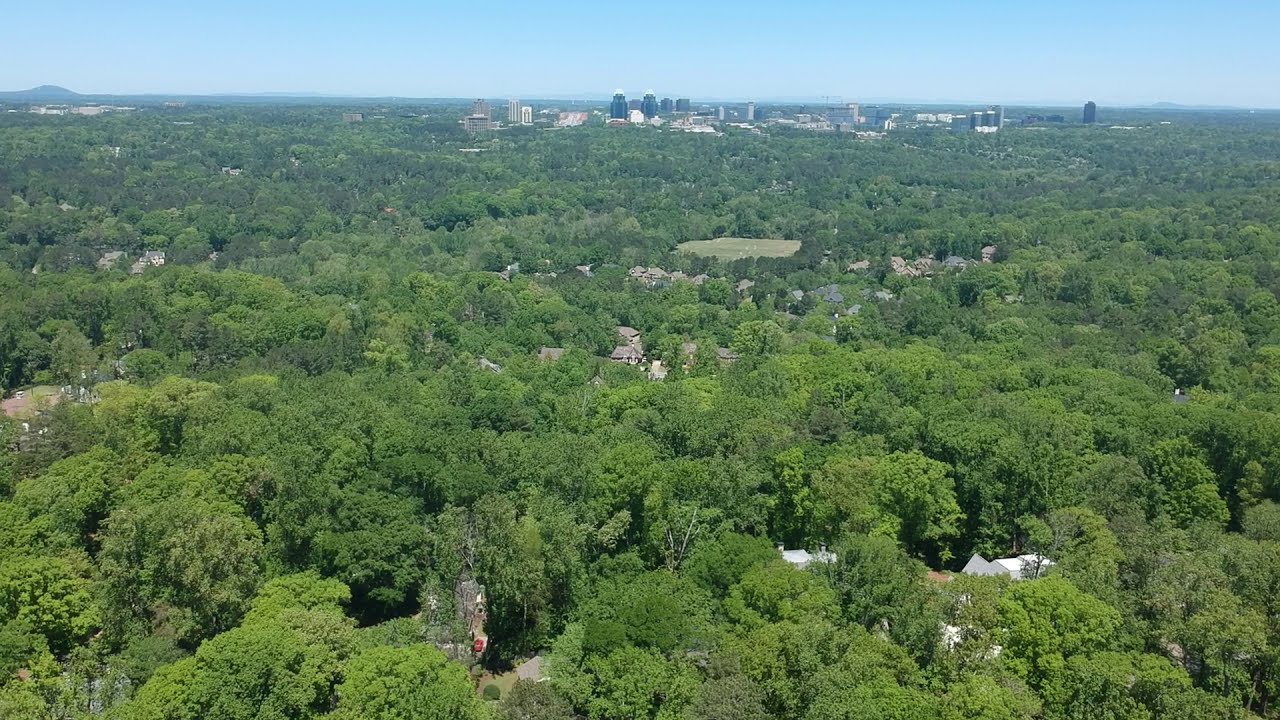The photograph captures an aerial view of a heavily forested area with tall, lush green trees extending across the landscape. Amidst the vibrant greenery, clusters of buildings are scattered at regular intervals. The buildings are predominantly white or gray, forming groups of five to ten structures each. In the central area, a distinct circular green field stands out, possibly a sports field, though its exact purpose is unclear. Towards the back of the image, a range of mountains rises on the top left, while the right side features a large open green area. Beyond this, a skyline of a modest city with several tall buildings, including prominent black and lighter-colored ones, can be seen. Interspersed among these are four round, tower-like structures hinting at industrial utility. The sky above is a bright, yet slightly blurry blue, devoid of visible clouds.